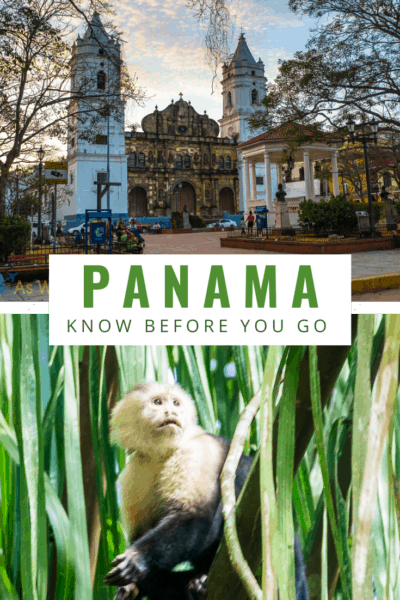The image comprises two distinct photographs placed vertically with a horizontal, white rectangular strip in between. Prominently displayed within the white strip is the word "PANAMA" written in large, green, capital letters with extra spacing between each letter. Directly below, in smaller font, the text reads "Before You Go."

The top photograph captures a picturesque church located in what appears to be a traditional Spanish or Latin American town square, possibly in South America. The church features two distinctive white steeples framing its brown facade against a clear blue sky. Scantily populated, the scene includes a few individuals and green shrubbery, preserving a serene, almost timeless ambiance.

The bottom photograph dramatically shifts in perspective to a close-up view of lush green grass. Nestled among the blades is a small monkey, likely a spider monkey, characterized by its white face, shoulders, and chest contrasted against its dark brown-black body. The monkey's visible left hand is raised and reaching, with its gaze directed towards the upper right corner, making a subtle connection to the photo above. The combined imagery showcases a palette dominated by various shades of green, complemented by blue, brown, and white, evoking a sense of natural beauty and cultural richness.